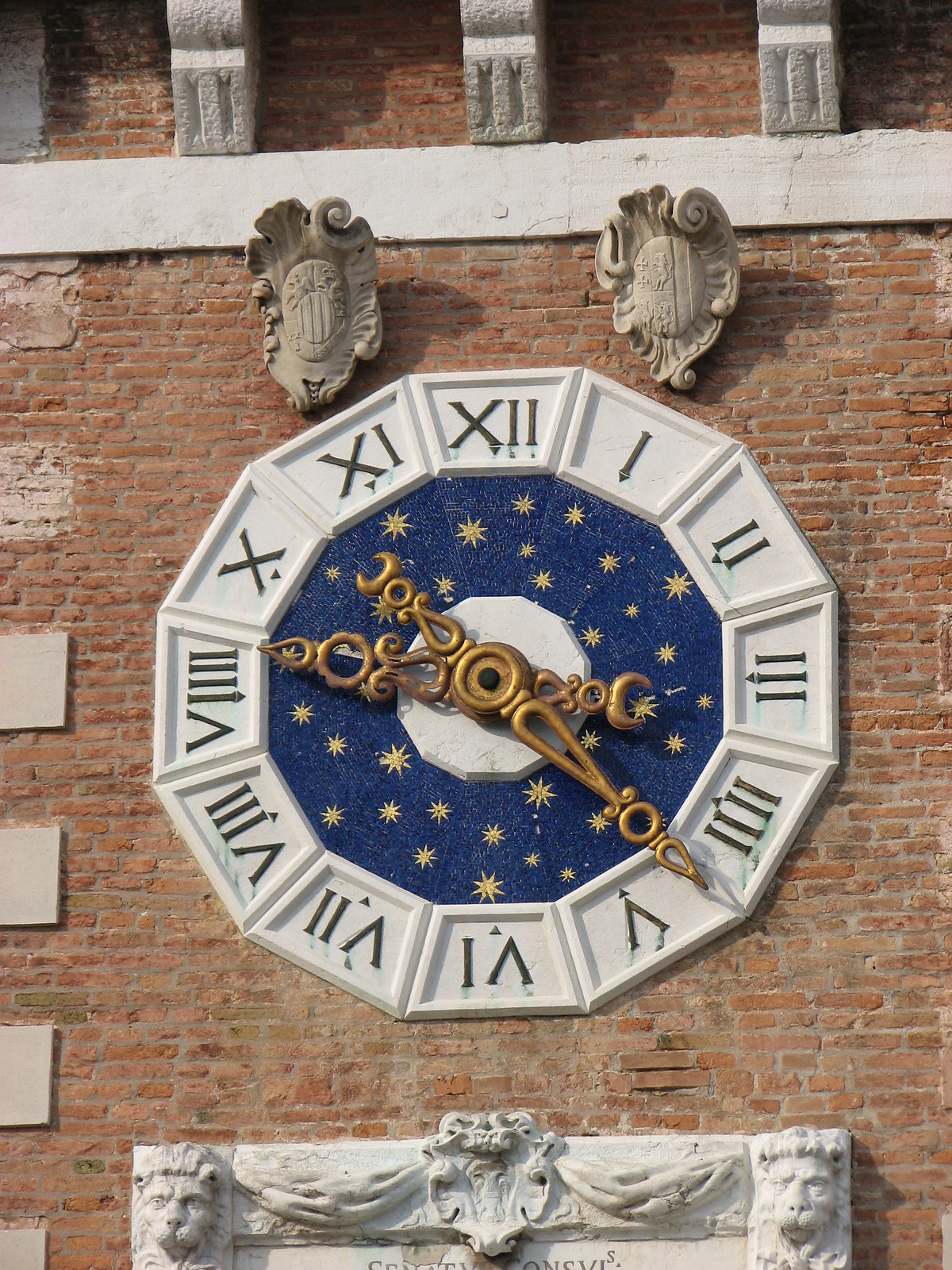The photograph showcases the exterior of a historic building characterized by its orange-brown brick façade with gray cement mortar. Dominating the scene is an ornate clock embedded into the wall, featuring gold-colored hands and Roman numerals (I to XII) in black against white stone sections. The clock face is set against a striking navy blue background adorned with gold stars. Above the clock, there is a row of tan-colored ornamental elements, while a line of white stone adorns the top of the structure. Below the clock, the building features intricately carved stone lion heads at the bottom left and right corners. Appearing to span across a gap—potentially over a monument—there is a partially visible inscription carved into the stone, hinting at the building's historical significance.